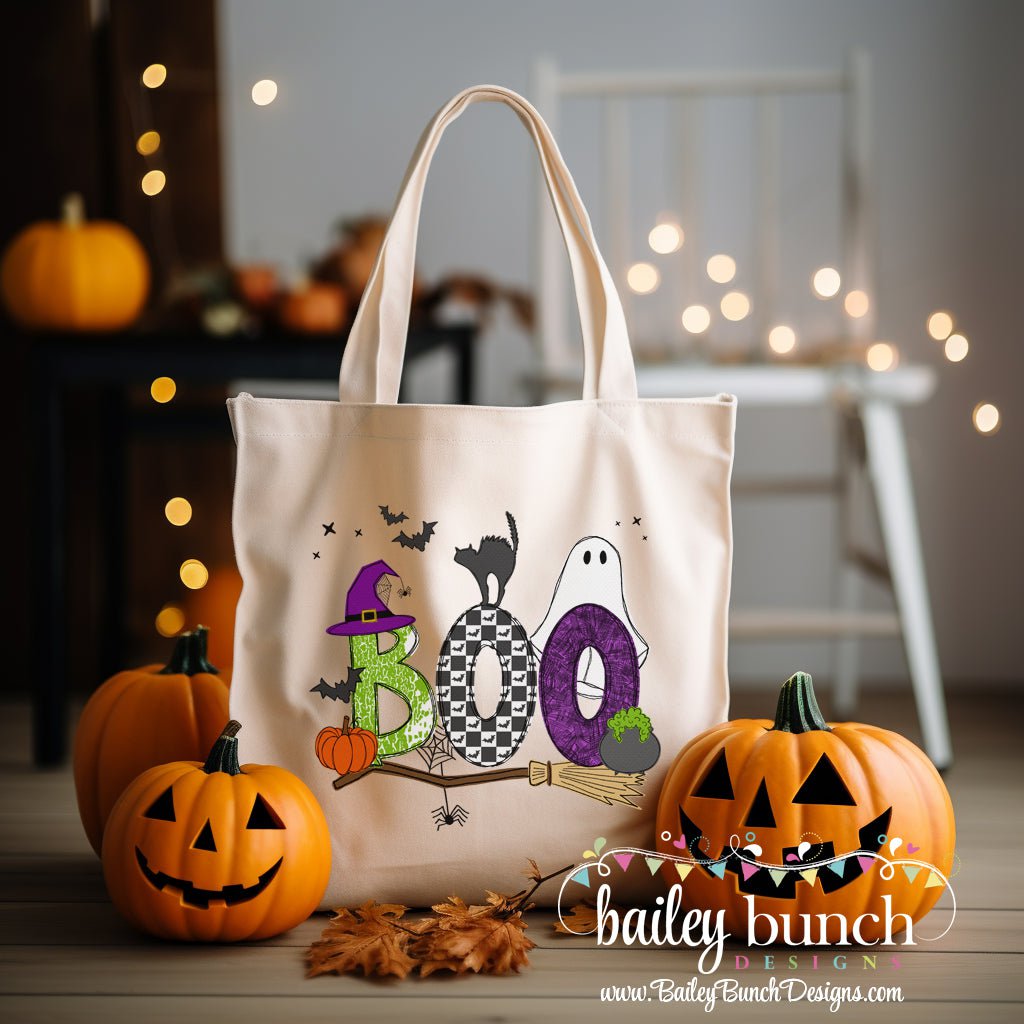In this detailed Halloween-themed image, a handmade off-white trick-or-treat bag is prominently displayed on a wooden floor. The bag is adorned with vibrant and festive decorations, including the word "BOO" in lively letters. The "B" sports a purple witch hat, the first "O" is a black and white checkerboard with a black cat perched atop, while the second "O" is purple with a ghost peeking from behind. Beneath the word is a witch's broom and small bats flutter around the bag. Additional features include a spider and a web nestled between the "B" and the first "O," and what appears to be a green cauldron near the ghost. Surrounding the bag are three small pumpkins and a few scattered autumn leaves, enhancing the seasonal ambiance. In the background, blurred festive lights adorn white chairs, adding a warm glow to the scene. The bottom right corner of the image bears the branding "Bailey Bunch Design" along with their websites, www.baileybunchdesigns.com and www.baileybunch.com.